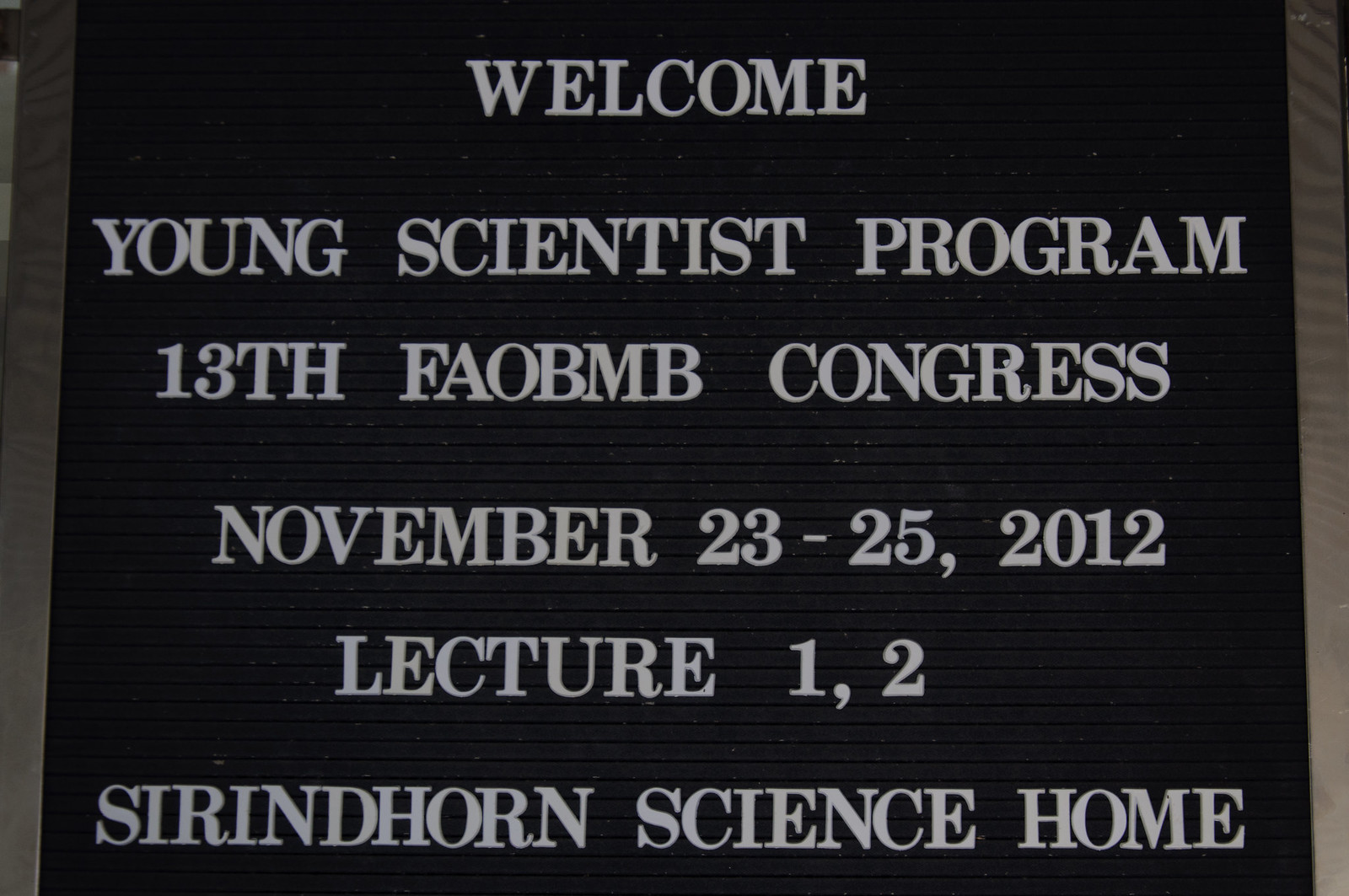The image is a simple color photograph of a nearly square, monochrome sign without a border. It features a black background and removable white capital letters, commonly used for customizable event signage often seen outside conference halls or lecture halls. The sign reads, "Welcome Young Scientist Program 13th FAOBMB Congress November 23-25, 2012 Lecture 1, Lecture 2 Sirindhorn Science Home." The setting appears to be an event sign placed at or near the entrance to a lecture hall, announcing details for an ongoing scientific program.